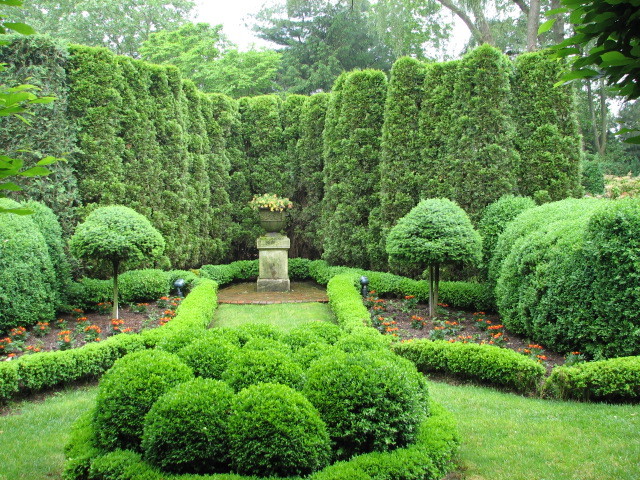The image depicts a meticulously maintained formal garden surrounded by a lush forest. The garden is filled with greenery, including both tall and short bushes, creating a serene natural ambiance. At the center of the garden is a square, stone pedestal serving as a planter, featuring vibrant yellow and orange flowers. This pedestal is encircled by low hedges and coned, mushroom-shaped small trees. The garden is structured with a mixture of mulch beds containing flowers, middle-sized bushes, and circular clusters of shrubs. The greenery is interspersed with small, round bushes numbering around a dozen, adding to the well-kept aesthetic. The background reveals towering, meticulously trimmed bushes, with taller trees visible beyond them. During daylight, the entire area showcases its vibrant plant life, while at night, decorative lights illuminate the stone centerpiece, enhancing its visual appeal. The landscape design, with its combination of pathways and various sized plants, presents an elegant and artistic composition.